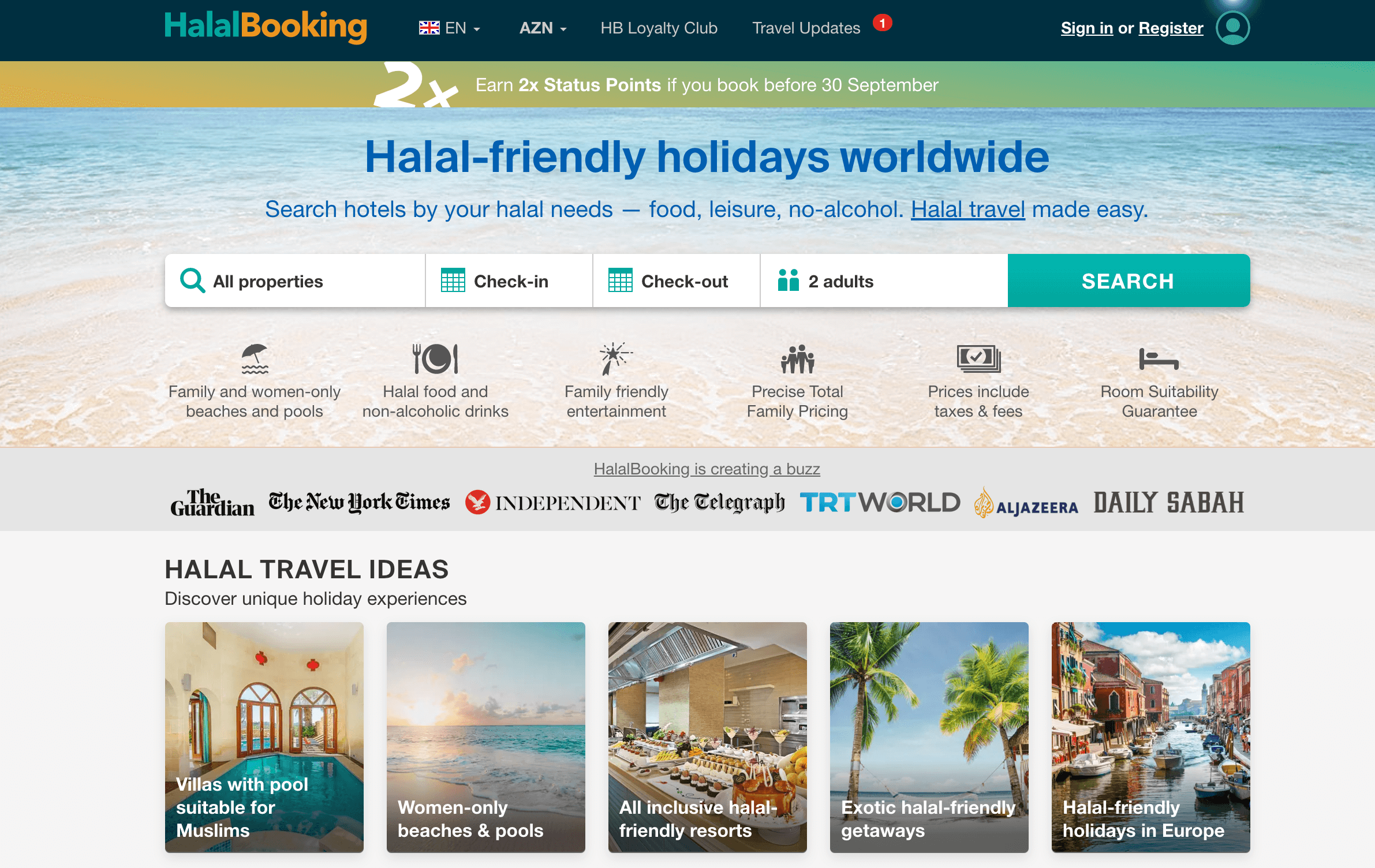This is a screenshot of a travel website tailored for Halal-conscious travelers. In the upper left-hand corner, the logo "Halal Booking" is prominently displayed, with "Halal" in teal and "Booking" in yellow. Adjacent to the logo, an Alaska state flag icon accompanied by the text "EN" signifies English language options. To the right of this, the currency "AZN" is displayed, followed by navigational links for "HB Loyalty Club" and "Travel Updates," the latter with a notification badge showing the number 1 in a red circle. On the upper right-hand corner, there is an option to "Sign In or Register."

Underneath, a promotional message alerts users to "Earn 2x Status Points if you book before 30 September." Below this, a tagline reads "Halal-Friendly Holidays Worldwide," followed by an underlined statement: "Search Hotels by your Halal Needs-Food, Leisure, No Alcohol, Halal Travel, Made Easy."

The central search interface consists of four distinct fields: "All Properties," "Check In," "Check Out," and "Two Adults" (which allows users to select the number of adults). A "Search" button is positioned to the right of these fields.

The website advertises several features from left to right: "Family and Women Only Beaches and Pools," "Halal Food and Non-Alcoholic Drinks," "Family-Friendly Entertainment," and "Precise Total Family Pricing," including taxes and fees with a sustainability guarantee.

Additionally, a section titled "Catching the Buzz" showcases endorsements from prominent publications such as The Guardian, New York Times, Independent, Telegraph, TRT World, Al Jazeera, and Daily Sabah. The page also highlights a section for "Halal Travel Ideas."